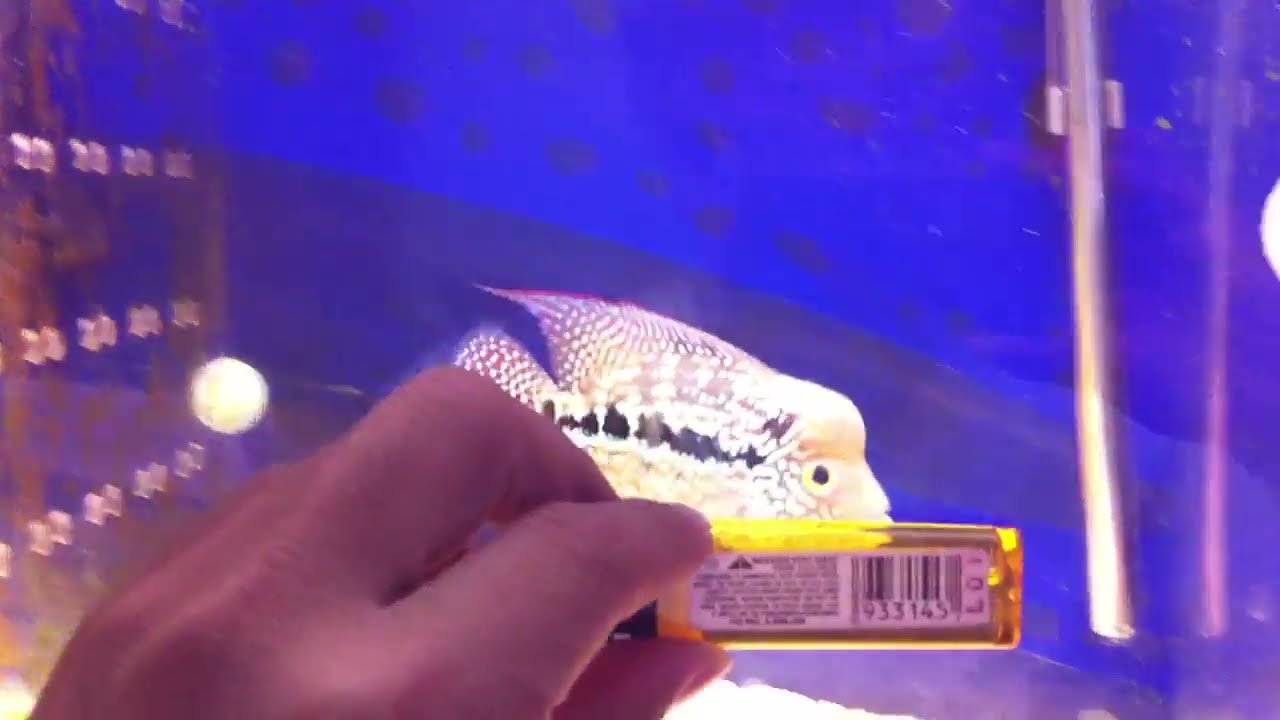The photograph features a chubby, cute fish with an array of vibrant colors, including a pale salmon base with black, white, and gray spots, accented with a hint of pink or peach. The fish has distinct, big yellow eyes with black irises and a notable bump on its forehead, reminiscent of certain types of goldfish. The fish, exhibiting shades of aqua blue, black, and yellow, swims gracefully in clear water within a small corner of the tank. The tank has a blue background, which might be external, creating a deep blue atmosphere. The floor of the tank is lined with small white stones and yellow stones. Featured prominently in the scene are two orangish-red bowls; one is real while the other is a reflection on the glass side of the tank.